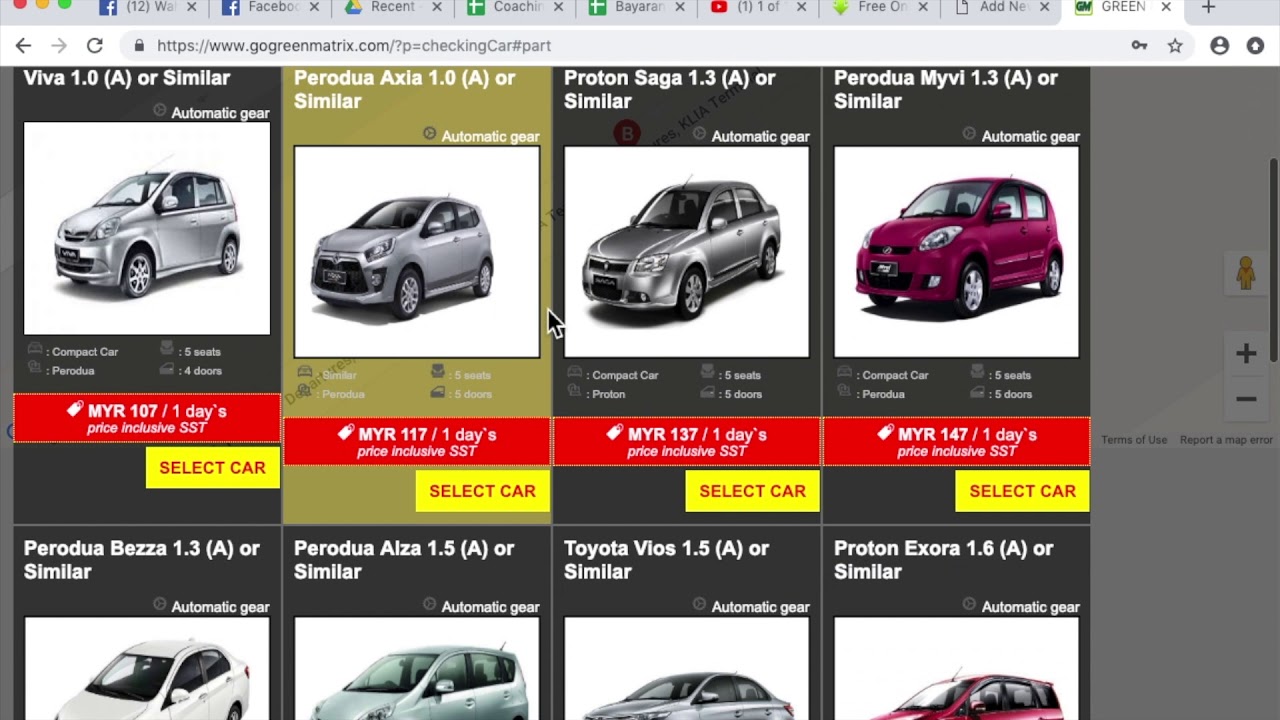The image displays a web browser with numerous open tabs. The highlighted tab has the word “Green” visible, indicating it belongs to the website “gogreenmatrix.com,” which appears to be focused on shopping for electric cars, possibly for rental. On the webpage, there are two rows of vehicle listings, though only the top row is fully visible. 

Each vehicle is photographed against a white background, with details outlined on either a black or gold background. 

1. The first car showcased on a black background is a silver vehicle described as "Automatic Gear via 1.0 (A) or similar." It's labeled as a compact car, specifically a "PERODUA," accommodating five seats and four doors. The price is listed as MYR 107 per day, including SST (Sales and Services Tax). A yellow "Select Car" button is present beneath each listing.

2. The second car is presented on a gold background, also a silver PERODUA but this time the model is specified as "Axia 1.0 (A) or similar." Like the first, it offers five seats but with an additional door, totaling five doors. The rental price for this model is MYR 117 per day, inclusive of SST. 

The price details for each vehicle are displayed in white text on a red background. Both listings suggest these are options for rental cars given the day rates and the “select car” prompt.